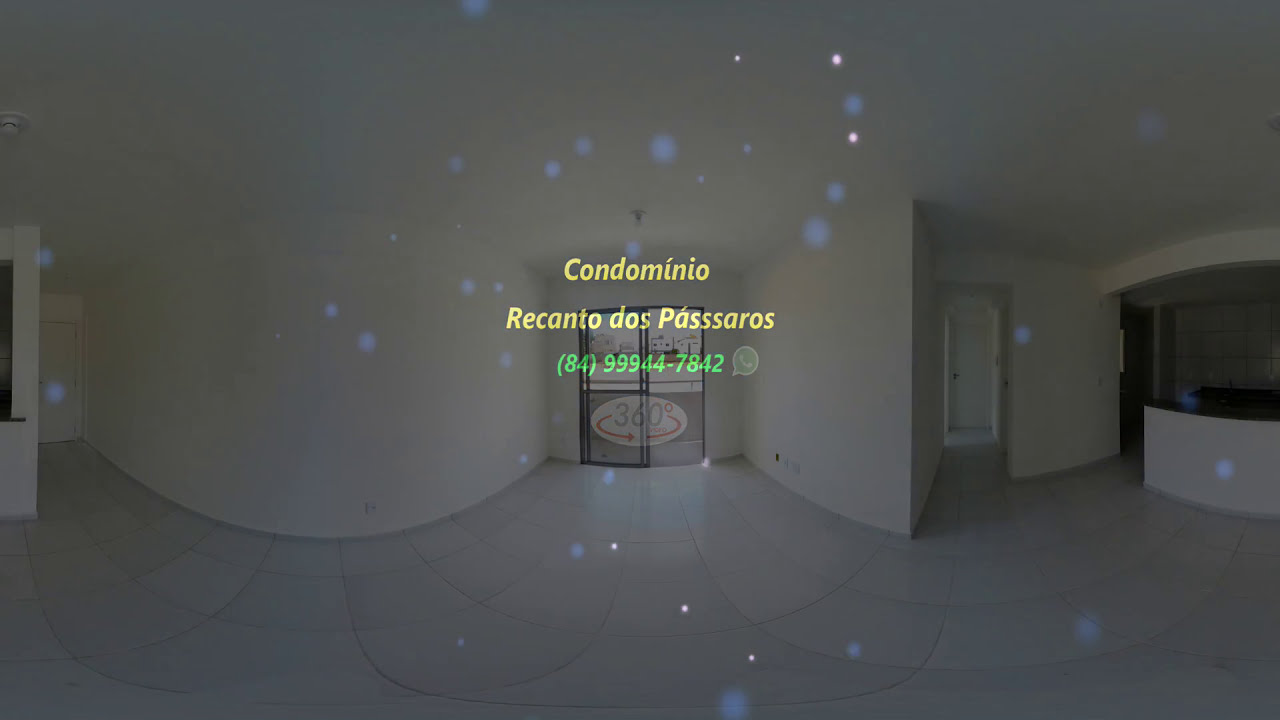The image depicts a dimly lit, underexposed indoor shot that appears to be a lobby area, potentially part of a business or an office space rather than a private residence. The space features white, antiseptic walls with significant curvature on both the left and right sides. In the center of the frame, mid-ground, and prominently overlaid in yellow text is the label "Condominio Recanto dos Pássaros," accompanied by a green phone number: "(84) 99944-7842," flanked by a semi-transparent WhatsApp icon. Below this text, a semi-transparent white oval displays "360" in light gray, encircled by a red arrow and circle. Additionally, the image includes a light gray tint overlay along with scattered blue and white dots. The area looks like a spacious lobby or living room, empty with a white-tiled floor and several doors: a sliding door leading to a balcony in the center, a corridor and door on the left, and another closed door on the right. To the far right corner, there appears to be an empty kitchen area. What might be a front desk is located on the right side of the space. This image likely serves a real estate or rental purpose, informing potential tenants or buyers about the property through the contact information provided.